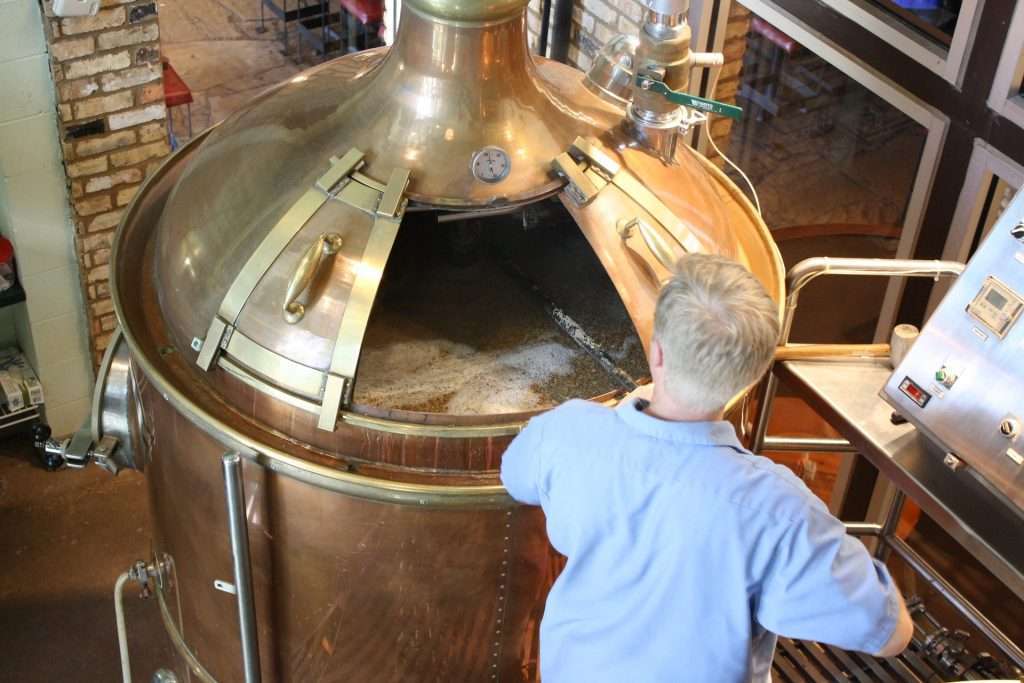The image captures an industrial-looking indoor setting featuring a large copper-colored contraption, presumably a beer brewing kettle. The photo is taken from a slightly above and angled perspective, highlighting the kettle's prominent features: a golden-brown metallic body, a built-in clock-like temperature gauge, sliding doors with handles on both sides, and tubes protruding from the top. A man with gray hair, wearing a blue shirt, is actively engaged with this kettle, using a long-handled tool, possibly a black stick or paddle, to mix the contents inside. The interior of the kettle appears dark, with a white foam visible, likely part of the brewing process. Surrounding the scene are various pieces of equipment with buttons and a neutral-toned brick wall adorned with some stools. To the right, there are floor-to-ceiling windows with black and white panes, allowing natural light to filter in. The overall palette of the image includes shades of black, white, gray, tan, off-white, brown, copper, and hints of blue and terracotta.